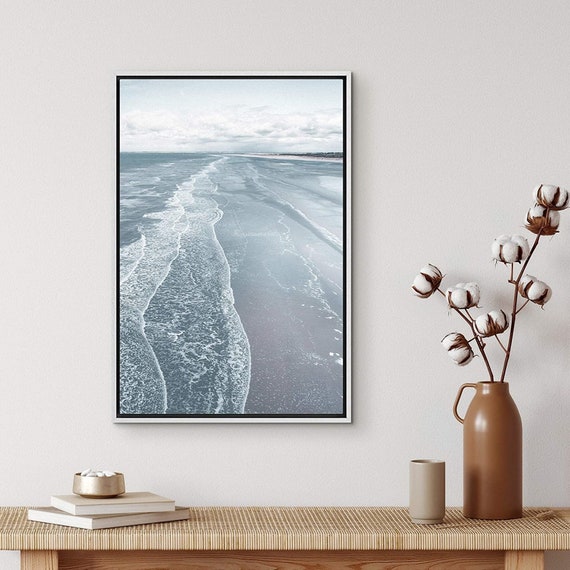The image features a serene, beige-toned room with a light gray wall serving as the backdrop. Central to the composition is a rectangular photo frame that captures a tranquil beach scene. The image within the frame depicts gentle waves lapping at a sandy shore, with a pale blue sky overhead, dotted by fluffy white and gray clouds. In the distance, faint outlines of land and trees are visible, adding depth to the scenery.

Beneath the framed photo, a modest wooden console table in a light brown hue, possibly bamboo or wicker, stretches horizontally. On the left side of the table, two books are stacked askew, topped by a small metal bowl. Centrally placed beside them, a sleek gray glass sits with understated elegance. To the right, a brown vase resembling a jug with a small handle holds decorative twigs adorned with white cotton puffs, offering a touch of rustic charm. The branches' brown stems contrast subtly against the white cotton, creating a harmonious blend of textures and colors. The overall arrangement on the table is completed with a small tray or cup near the vase, all combining to create a thoughtfully curated and visually soothing decorative ensemble.